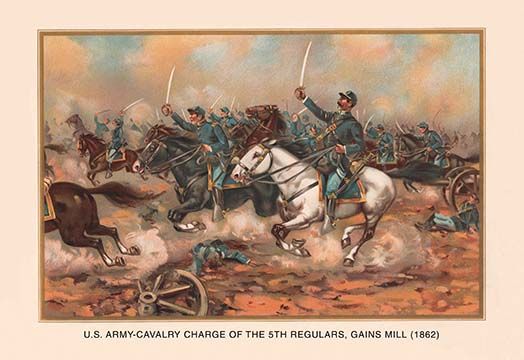The image depicts a vivid and chaotic battle scene titled "U.S. Army Cavalry Charge of the 5th Regulars, Gaines Mill, 1862," as labeled beneath the painting. Dominating the scene are numerous Union cavalry soldiers dressed in blue uniforms, actively engaged in combat, brandishing swords in their left hands while riding on horseback. The central figure, prominently placed, is astride a striking white horse, flanked by another rider on a black horse. Most of the horses are brown. The battleground is littered with fallen soldiers and broken equipment, including parts of cannons, some shattered and others still intact, as well as a broken wagon wheel in the bottom left. The ground is predominantly rust and brown-toned, adding to the chaos and drama of the scene. Billows of smoke—possibly from cannons—intermingle with the blue sky and clouds, enhancing the sense of turmoil. In the background, more cavalrymen can be seen charging forward. The painting is surrounded by an off-white tan mat and frame, suggesting it might be displayed in a museum.